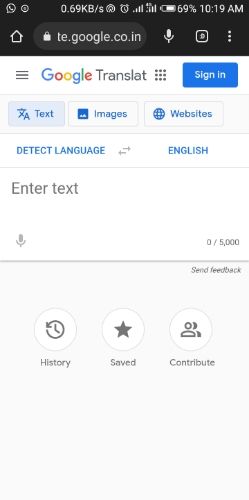Screenshot of Google Translate page, showing various icons in the notification status bar at the top. There is a missed call icon, a data usage indicator showing 0.69 KB/s, a 4G signal indicator, and a battery level at 69%. The time displayed is 10:19 AM. 

The Google Translate interface offers three main options: entering text manually, uploading an image, or inputting a website link. The current setting is configured to translate text into English. Below this, there are three additional options labeled History, Saved, and Contribute. Overall, the image captures a rectangular interface of the Google Translate page with multiple functionalities visible.